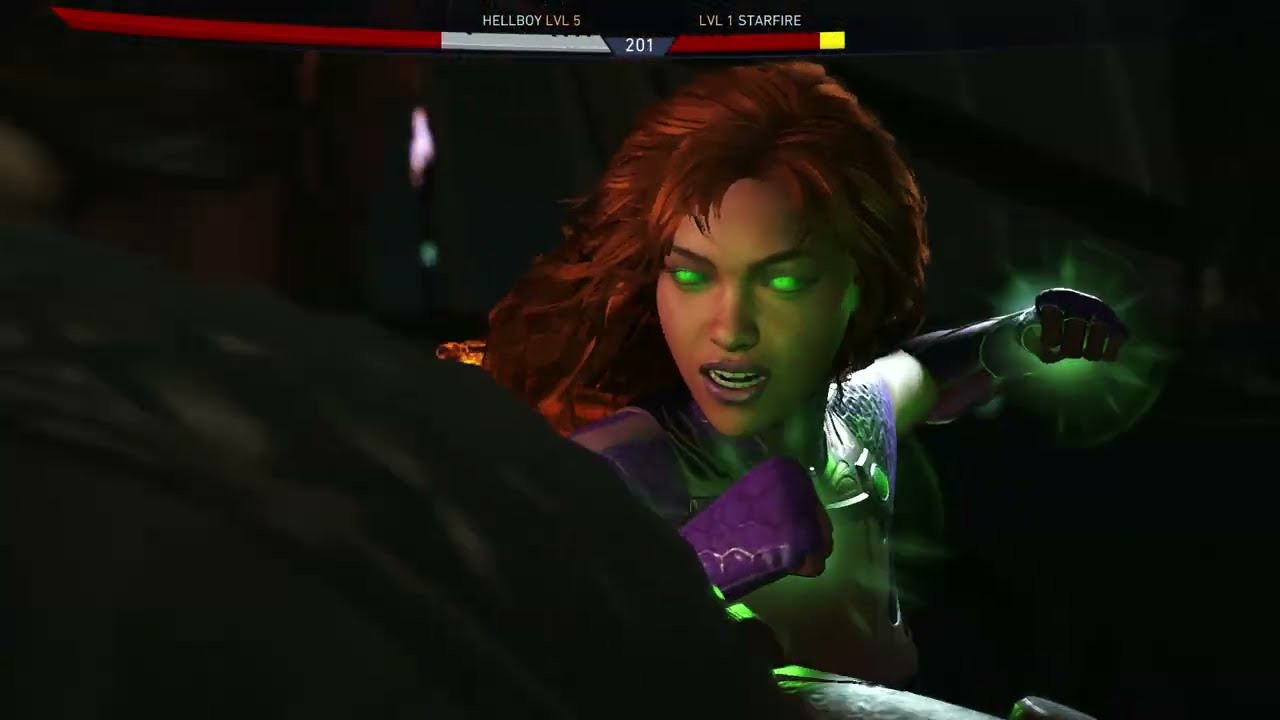The image is a still from a video game featuring a dynamic fight scene. Dominating the center is a digital depiction of a human-like female character with auburn hair and glowing lime-green eyes. Her skin has a peach complexion, and she is dressed in intricate purple and gray armor. A striking feature is her left fist, cocked back and surrounded by a green light indicating power, suggesting she’s about to punch an unseen opponent. Above her, a vibrant banner displays the names and levels of the characters in combat: "Hellboy Level 5" on the left side with a red, gray, and yellow bar, and "Starfire Level 1" on the right side with a blue and silver bar. Both of these status bars have the number "201" prominently displayed, adding to the immersive experience. The scene bears a resemblance to a classic "Mortal Kombat" style video game, with the attention to detail in the character's depiction and her poised stance ready for battle.